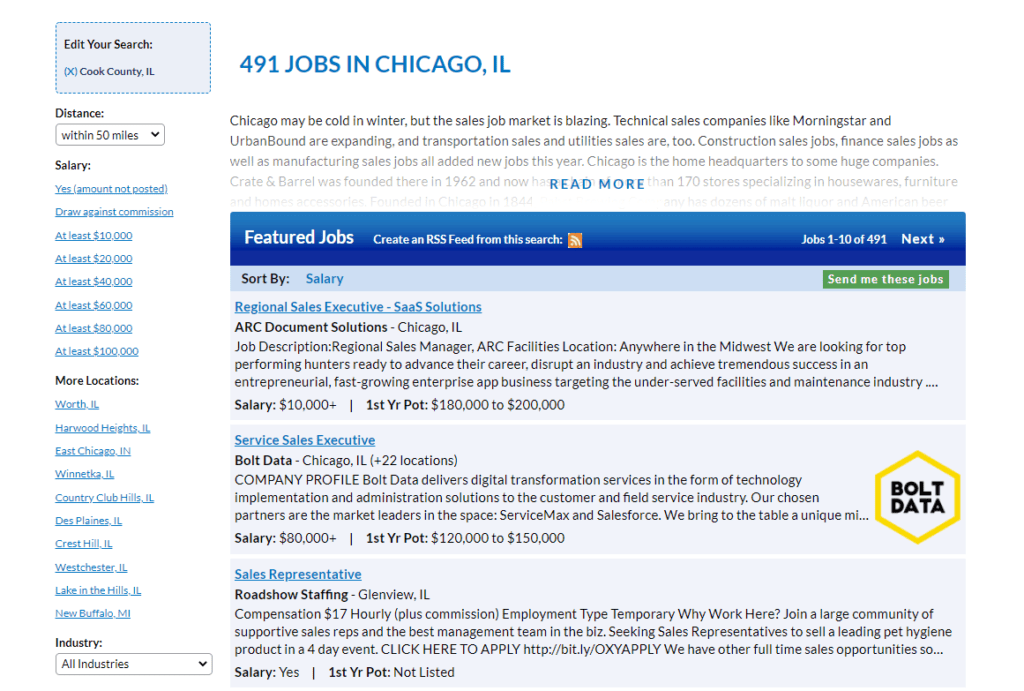The screen capture showcases a job board website displaying a total of 491 job listings in Chicago, Illinois. At the top of the page, there's an option to create an RSS feed from the current search query. Featured job titles include "Regional Sales Executive," "Service Sales Executive," and "Sales Representative," among others. Detailed information is provided for each job, including salary ranges and job descriptions. 

The search is refined to Cook County, Illinois, and encompasses a radius of 50 miles. Users can sort job listings by various salary categories, such as at least $10,000, $20,000, $40,000, $60,000, $80,000, and $100,000 per year. Additionally, the website offers the option to search for jobs in other nearby locations within Illinois. The layout allows users to scroll through job listings efficiently until they find a position that meets their criteria.